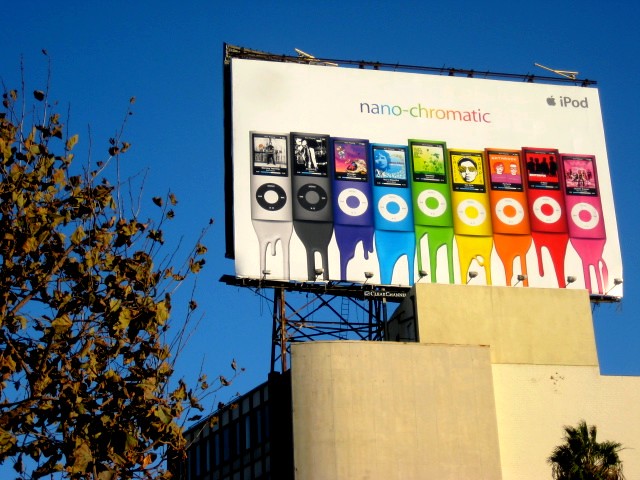The image depicts a vibrant billboard advertisement set against a clear blue sky. On the left-hand side, a tree with very dry leaves stands prominently. In the bottom right-hand side, there is part of a building with the billboard mounted on its rooftop. The advertisement itself features a white background, displaying nine iPods arranged in a gradient from left to right: white, gray, purple, blue, green, yellow, orange, red, and pink. Each iPod appears to be dripping its respective color. Above the iPods, in corresponding colors, is the word "nano-chromatic." In the top right-hand corner of the billboard, the iconic Apple logo and the word "iPod" are displayed. Additionally, the very top of a palm tree is visible in the bottom right corner of the image.